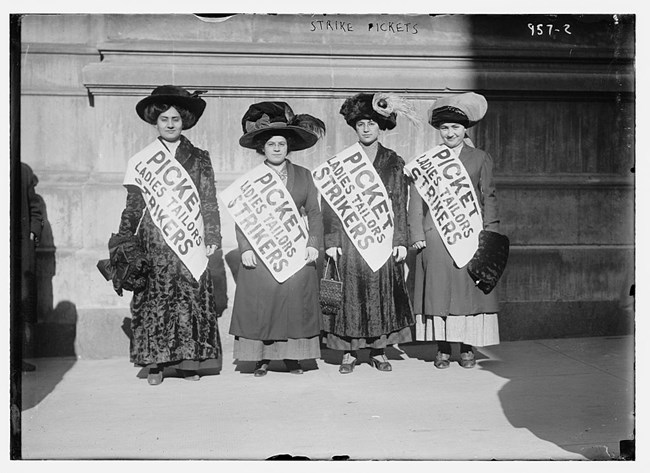A horizontally aligned, black-and-white photograph showcases four women, likely from the early 1900s, demonstrating their solidarity as picket ladies and tailor strikers. Each woman wears a large, decorative hat—some adorned with feathers or lace—and diagonally across their shoulders, they sport sashes that read "Picket Ladies Tailors Strikers". The women are dressed in coats and dresses, with the one on the far left standing out in a striking cheetah-print fur coat. They stand poised and confident against a stone wall, which appears light gray on the left and middle side and dark gray on the right side. Carved prominently at the top of the wall are the words "Strike Pickets", while the upper right corner of the wall features the graffiti-like writing "957-2". They stand on a sidewalk outside the building, casting shadows on the ground, each looking directly at the camera.